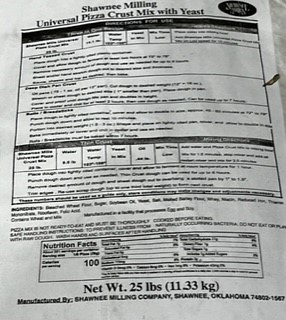This image, a somewhat low-quality and small photograph, appears to capture a product label laid on a slightly wrinkled piece of paper over a gray background. The label is from Shawnee Milling, clearly spelled out in bold black text, with the product identified as "Universal Pizza Crust Mix with Yeast." Although many of the finer details and additional text are too small to read, some critical information is visible. At the bottom of the label, the nutritional facts box prominently displays "100 calories per serving." Further down, larger, bold black text notes the net weight as "25 pounds (11.33 kilograms)." The overall appearance suggests that this is an information sheet for the Shawnee Milling company's pizza crust mix product.